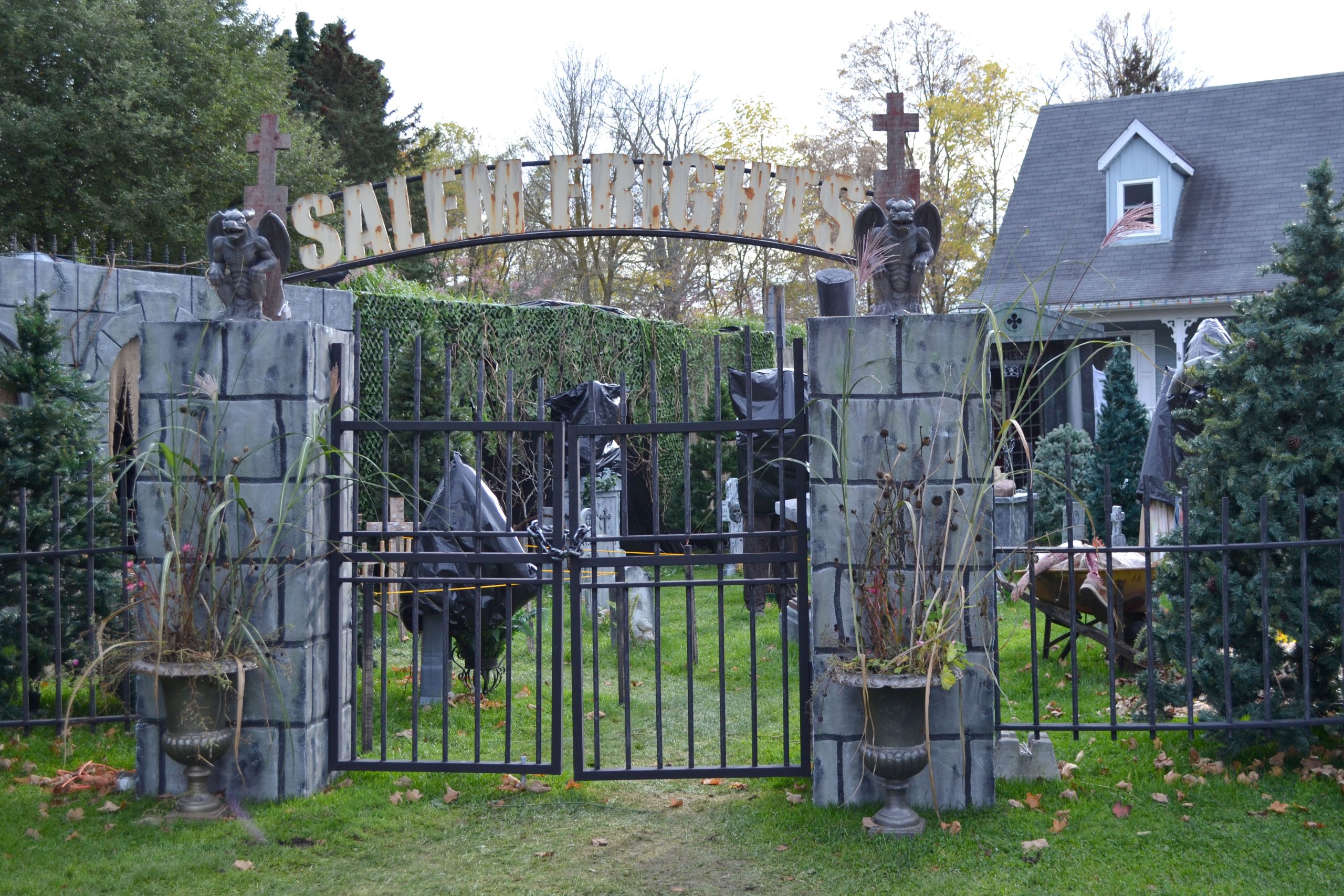In this image, a haunted house setting, presumably arranged for Halloween, is illustrated. The entrance features imposing stone pillars flanked by metal gates and adorned with formidable gargoyle statues perched atop each pillar. Above the wrought iron gates, which are rusted yet predominantly white, an arch sign reads "Salem Frights," flanked by crosses on either side. At the base of the pillars, there are flowerpots, though their plants appear more like weeds. The house visible behind this eerie setup resembles a New England cottage with a gray, slightly tiled roof and white trim. In the backdrop, one can discern a tall fence overgrown with grass and moss, along with some tombstone-like structures, enhancing the cemetery-like atmosphere. The yard still boasts green grass despite a few barren trees hinting at the fall season. A couple of trees stand stark against a pale sky, contributing to the somber and spooky ambiance of the scene.